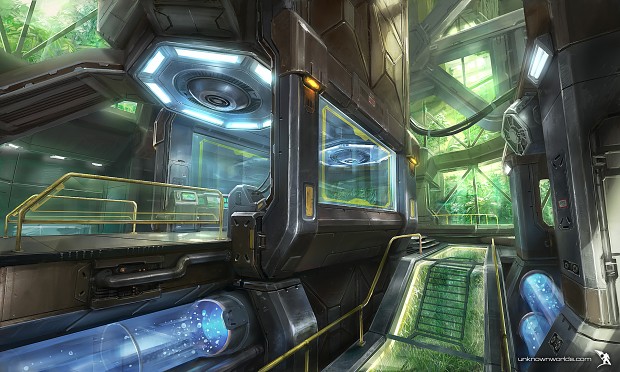The image depicts a detailed, futuristic sci-fi urban scene, likely a computer-generated illustration set in a large, indoor environment with distinctive architectural features. Central to the composition is a green walkway with a yellow railing, leading towards multiple tiers of buildings and additional staircases. Flanking the walkway are bright blue, transparent tubes filled with a bubbling liquid, suggesting some sort of futuristic water or liquid transport system. The scene is filled with numerous lights, possibly 60 to 70, illuminating the intricate metal and glass structure. The walls are made of metal with extensive use of glass, allowing visibility through tall, multi-story windows that offer a glimpse of lush green foliage outside. There's an abundance of lighting, including octagon-shaped ceiling lights with circular centers, creating a vibrant and otherworldly atmosphere reminiscent of an advanced spaceship interior. Additionally, the image features a website at the bottom, "unknownmortals.com," suggesting perhaps the source or inspiration for the artwork.